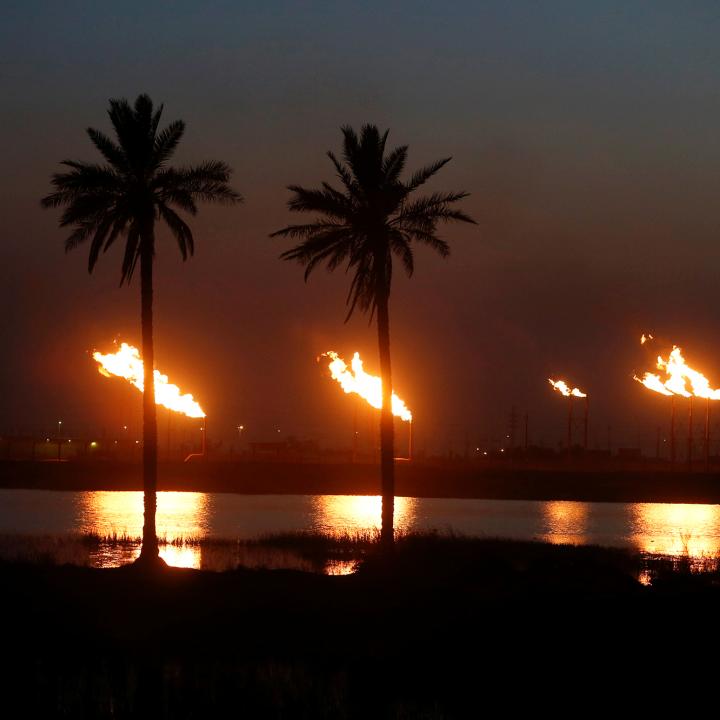This nighttime photograph captures a striking contrast between the natural and industrial landscape. The bottom fourth of the image is entirely black due to the absence of light, giving the foreground an impenetrable darkness. Rising from this obscured ground are two towering palm trees, distinctly silhouetted against the dark sky. One palm tree is positioned closer to the left side of the image, while the other stands almost perfectly centered. The trunks of these trees ascend high, with their fronds nearly reaching the top of the photo.

Behind the imposing palm trees lies a body of water that mirrors the intense light from the industrial background. Across this waterway, chimneys from a refinery or factory emit bright, fiery flames. These flames are prevalent and striking, especially noticeable on the right side where three stacks are clustered together, their flames intertwined. Additional chimneys in the central and left portions of the image also spew fire, creating a horizontal line of industrial activity that illuminates the hazy night sky. The sky itself is a mix of black and varying shades of dark blue and gray, adding to the overall somber yet dramatic atmosphere of the photograph.